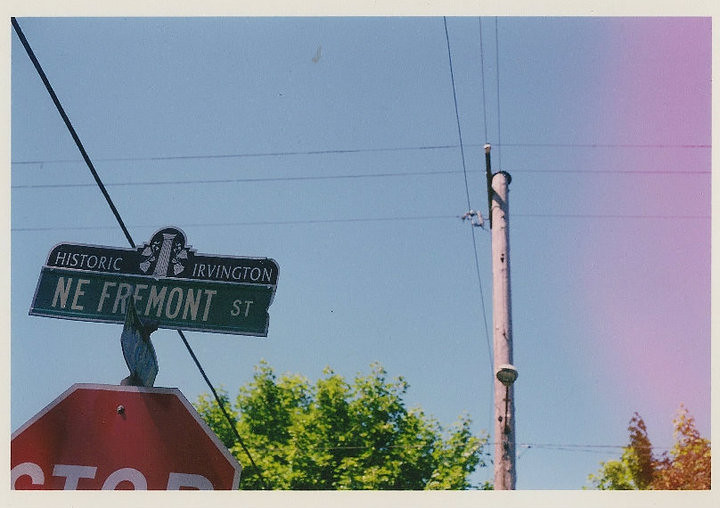This outdoor photo captures a vibrant and filtered street scene under a clear, cloudless sky that transitions from blue to a purple hue on the right side. Dominating the scene is a power pole with a light emanating from it, accompanied by six power lines stretching across the image. In the lower left-hand corner, the top part of a stop sign is visible, with an adjacent, unlegible street sign positioned above it. Additionally, another green street sign reads "Northeast Fremont Street," topped by a black or dark blue sign with white lettering that states "Historic Irvington." Two trees flank the power line, adding a touch of nature to the urban landscape.